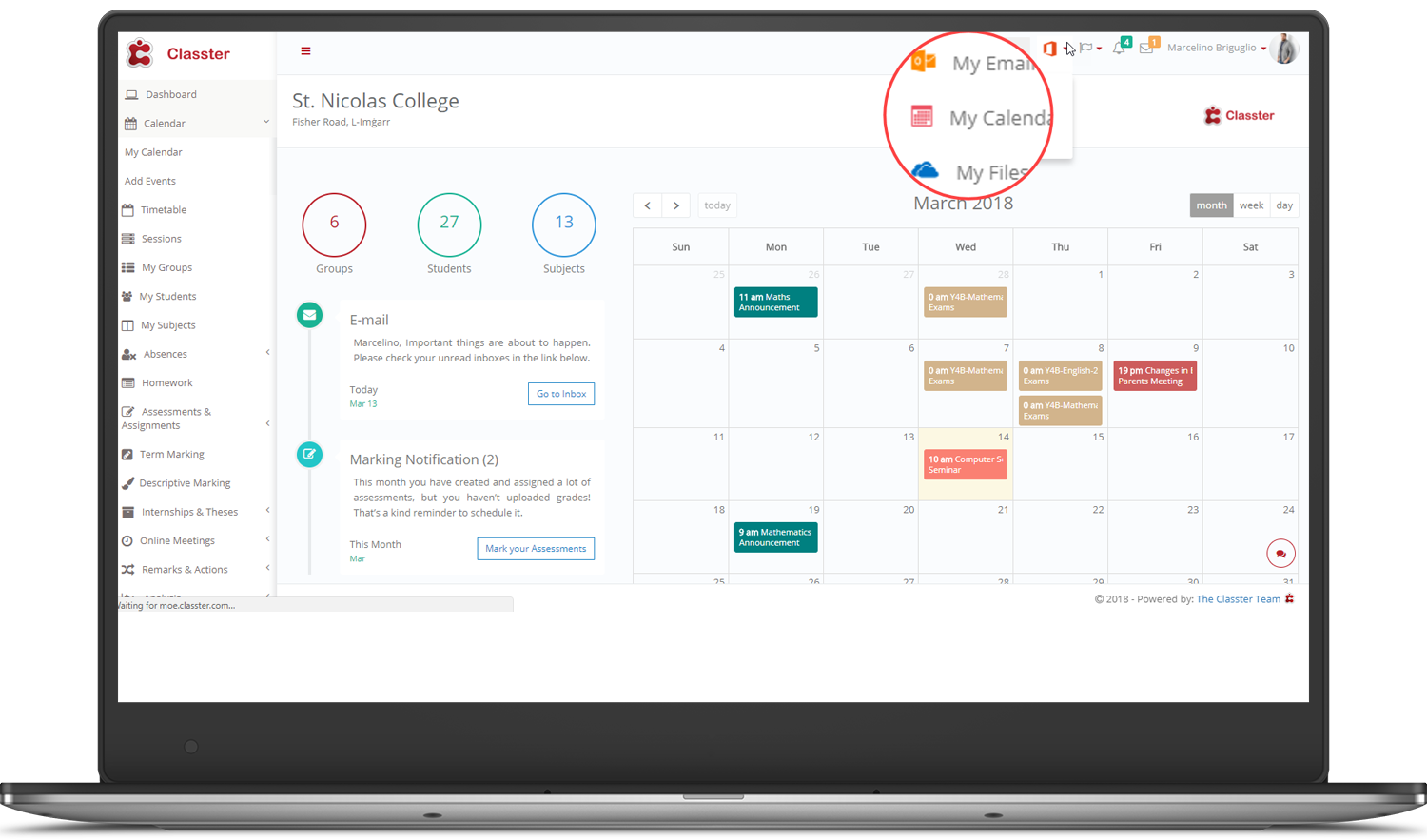This detailed screenshot showcases the interface of a college dashboard, likely from St. Nicholas College. In the top right corner, the word "Cluster" is prominently displayed in red letters. A sidebar on the left provides various navigation options including Dashboard, Calendar, My Calendar, Add Events, Timetable, Sessions, My Groups, My Students, My Subjects, Absences, Homework, Assignments, and Team Marketing.

Central to the screenshot, "St. Nicholas College" is highlighted in large letters. Below this heading, there are circular icons labeled Groups, Students, and Subjects, each with corresponding numeric values. To the left, indicating the current screen view, is the Calendar section. This calendar displays upcoming events for the user, color-coded in shades of green, beige, and red, suggesting different categories or priorities.

Additionally, there is a zoomed-in portion showing a dropdown menu activated by a caret toggle button. This zoomed-in menu includes options such as My Email, My Calendar, and My Files, likely providing guidance on navigating the dashboard effectively.